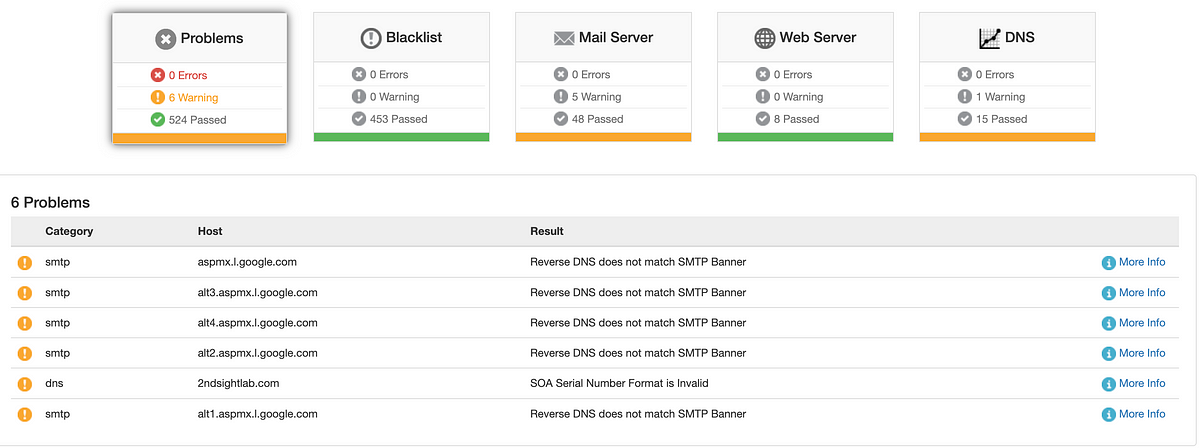This image depicts a detailed web management panel tailored for web developers and IT specialists, consisting of five distinct panels aligned horizontally at the top, each with a corresponding colored bar at the bottom. The first, third, and fifth panels feature orange bars, while the second and fourth panels are marked with green bars. The panels are labeled as follows: "Problems," "Blacklist," "Mail Server," "Web Server," and "DNS."

Each panel displays three icons underneath them, representing "Errors," "Warnings," and "Past Checks." The "Problems" panel is currently selected, revealing it contains 0 errors, 6 warnings, and 524 past checks. Below this selection, a detailed table is presented outlining the specific issues.

This table lists six problems, with column headers reading "Category," "Host," and "Result." Each entry in the "Category" column is labeled "SMTP" in lowercase, accompanied by a yellow circle with an exclamation mark to the left, signaling an issue. In the "Host" column, various hosts are listed such as "aspmx.l.google.com," among others with similar formats, but each entry is unique.

The "Result" column lists specific problems encountered:
- The first four entries state: "Reverse DNS does not match our SMTP banner."
- The last entry states: "SOA serial number format is invalid."

To the right of each result, there is a light blue circle containing a lowercase "i" for "information," and adjacent blue text reading "More Info," indicating additional details are available for each issue.